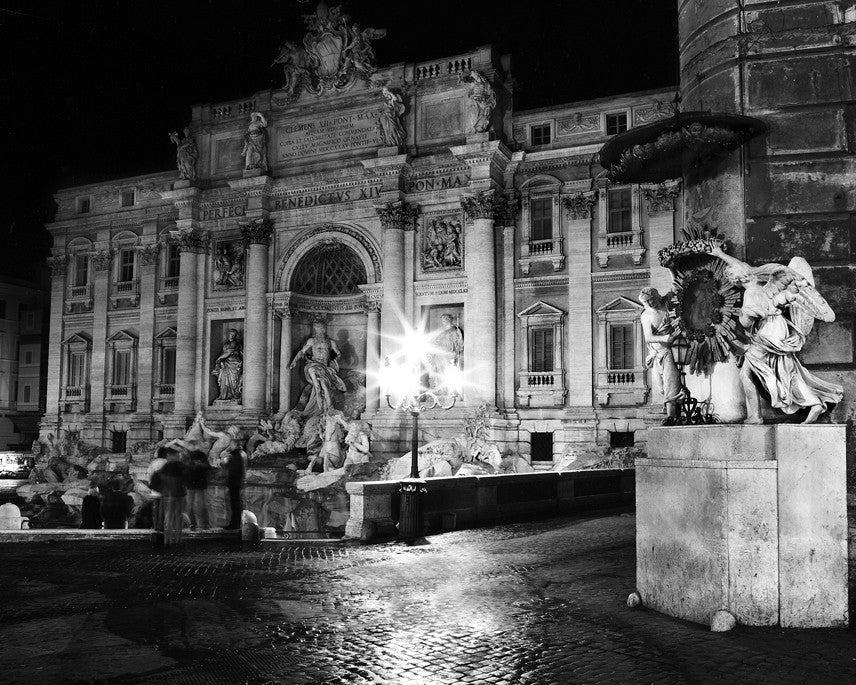This black-and-white photo depicts an old European palace, possibly reminiscent of the Trevi Fountain structure in Rome, which serves as the backdrop of the image. The palace, constructed predominantly from stone, features several grand columns, numerous intricate statues, gargoyles, and archways, showcasing highly ornate and historic architectural details. 

Against the dark, night-time setting, an ornate chandelier-style street lamp illuminates the scene, casting light onto a wet, cobblestone path that leads towards the structure. The palace itself is adorned with inscriptions that are difficult to decipher in the image. Prominently above one archway is an inscription that seems to read "Benedict XIV" alongside other text that is less clear.

In front of the palace is an elaborate fountain with multiple sculptural elements, featuring angels, demons, and various water spouts. A significant statue to the right of the image shows two figures flanking an insignia, possibly a dark star, placed on a massive white base. There is a small, somewhat blurred group of people near the fountain, providing a sense of scale while reinforcing the still-life quality of the photograph. The entire setting creates a luminescent and timeless atmosphere, highlighting the historic grandeur of the scene.